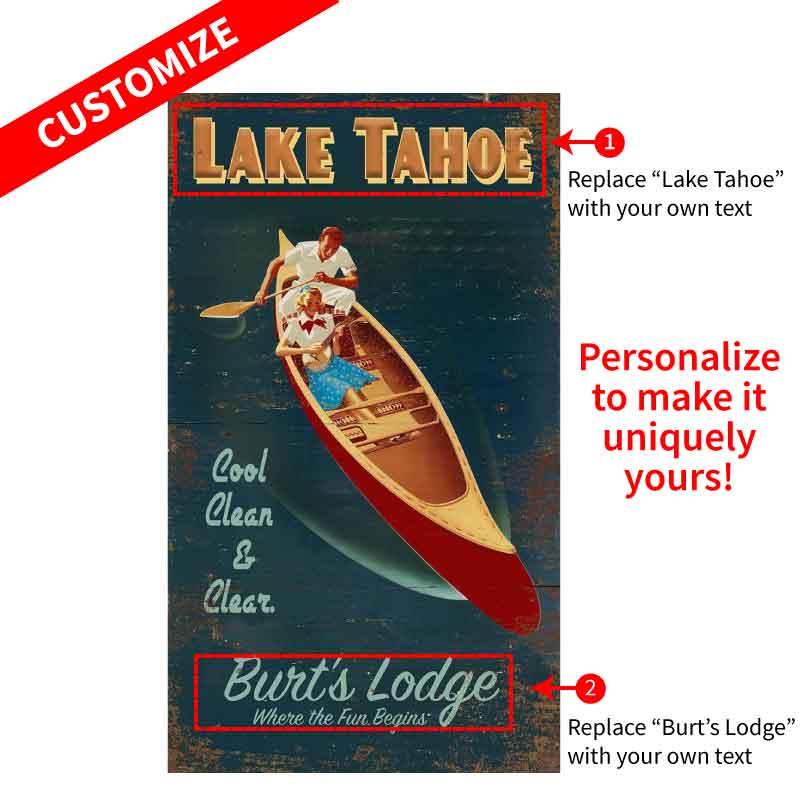This detailed poster demonstrates how businesses can customize their advertising. At the top left, there's a red banner with "Customize" written in white letters. Below it, the title "Lake Tahoe" appears in brownish letters, accompanied by an indication to replace this text with personalized content, marked as number one with an arrow pointing to it. To the right of the poster, in red lettering, it states, "Personalize to make it uniquely yours."

The main image in the center features a serene scene of two people in a red canoe on a lake, with an orangey-beige background. The man, seated in the front, is paddling and wearing a short-sleeved white collared shirt. The woman, sitting behind him, is playing a lute or a ukulele and is also dressed in white. Below the canoe, in a red rectangle with light blue lettering, the text reads, "Burt's Lodge, where the fun begins." This part of the text is highlighted as replaceable, with a small circle to the right of the poster marked as number two, indicating one can switch "Burt's Lodge" with their own text.

Additionally, there is text at the bottom of the poster in black letters instructing to replace "Burt's Lodge" with your own text. The overall design encourages customization of each text element to tailor the advertisement for individual businesses, providing a template for creative and personal adjustments.